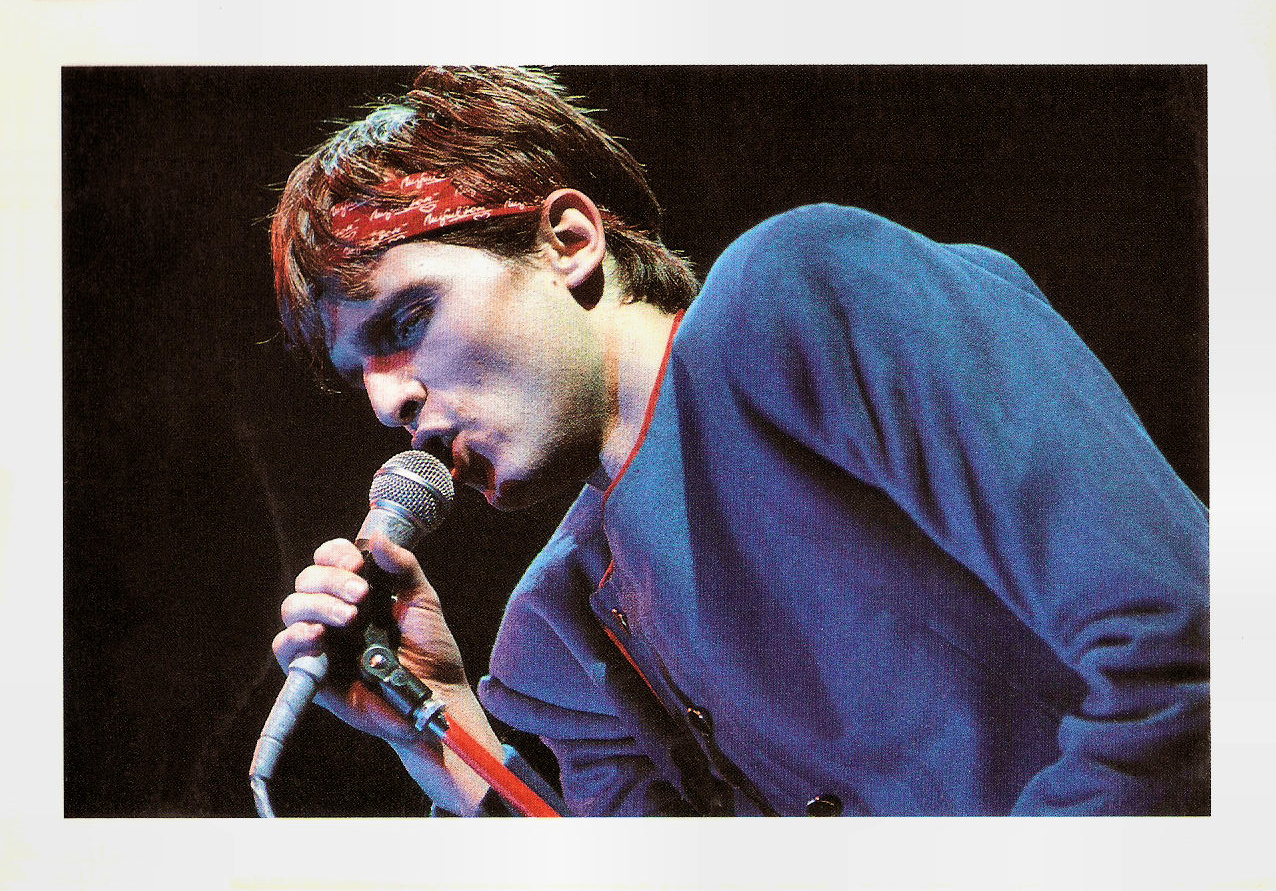This is an image of a young singer performing on stage, captured in a detailed close-up. He has short brown hair partially covered by a red and white bandana that drapes over his forehead and around his head. He is wearing a distinctive blue jacket, notable for its orange lining, collarless design, and offset black buttons. The jacket is made of a soft, felt-like material and features a red border that matches both the bandana and the red microphone stand he's gripping with his right hand. His angular face is dimly illuminated against a completely black backdrop, with the light highlighting his concentrated expression as he leans forward, eyes partially closed, lips pursed around the black microphone. The intimate and isolated setting emphasizes the earnestness of his performance.